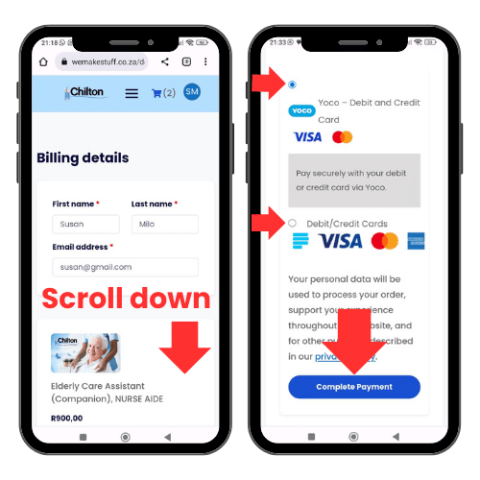The image showcases two smartphones placed side-by-side, each enclosed in a black case with visible side buttons. 

On the left smartphone's screen, a webpage from "wemakestuff.co.za/d" is displayed. The top section features a pale blue bar reading "Chilton" alongside a cart logo. Beneath this, the page asks for billing details, including first name, last name, and email address. Overlaid on this screen in red text are the words "scroll down," accompanied by a downward arrow. Further down, it includes text indicating "elderly care assistant nurse aide."

The right smartphone's display is focused on a payment processing page. The page displays the Visa card logo and mentions "Yoko debit and credit card," indicating that users can "pay securely with your debit or credit card via Yako," which is spelled "Y-A-C-O." It lists various cards accepted, including American Express, Visa, and MasterCard, and states that "your personal data will be used to process your order." The page ends with a "complete payment" button. Red arrows are strategically placed: one pointing to a bullet point in front of the first Visa logo, another targeting an unfilled circle in front of the second logo, and a final arrow pointing down at the "complete payment" button.